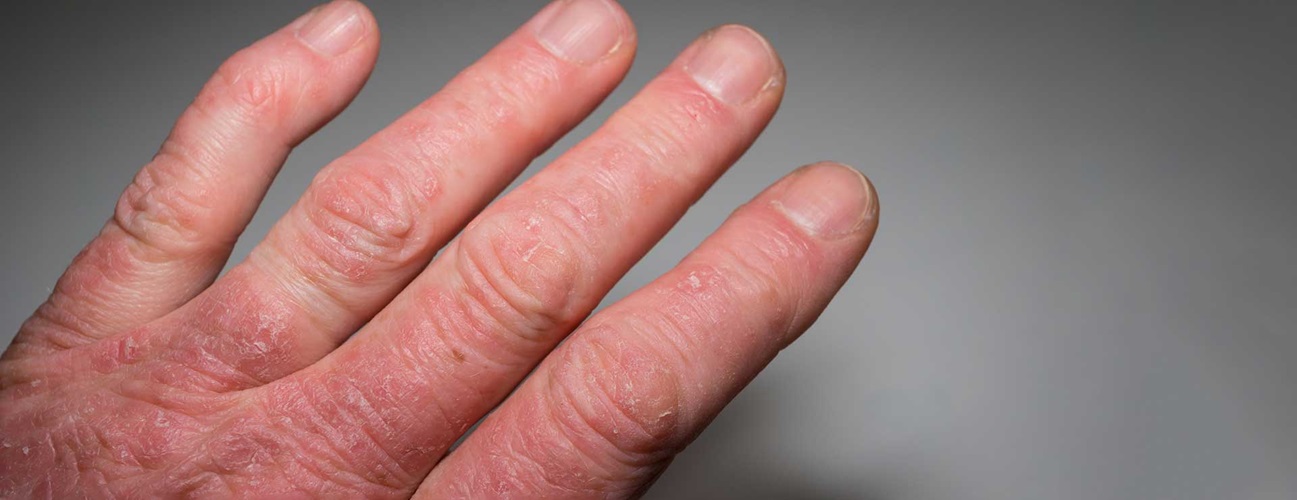This image features a detailed view of a white man's hand against a light gray background. The hand emerges from the bottom left-hand corner of the frame, extending diagonally towards the top center. The visible portion of the hand includes four fingers and a bit of the back of the hand, with the fingers slightly bent and outstretched. The skin displays numerous wrinkles and crease marks, particularly concentrated around the knuckles and between each joint. The knuckles have a reddish hue with noticeable white flakes indicative of dry skin. The fingernails are short and trimmed. Notably, the pinky finger towards the upper left of the image is slightly more bent than the other fingers. Overall, the hand shows signs of roughness and dryness, especially on the knuckles and towards the lower part of the back of the hand.